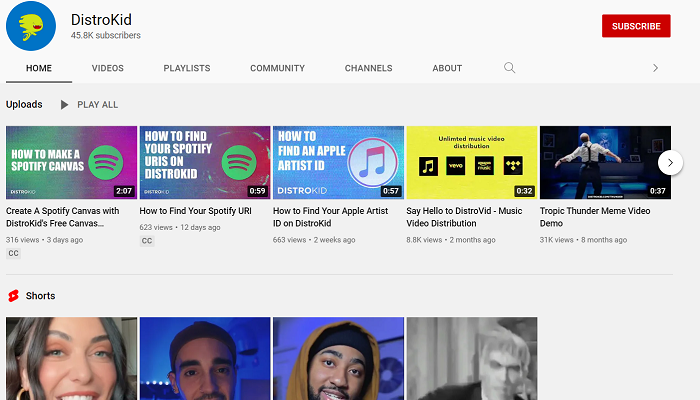This is a detailed screenshot of a web page, specifically a user interface that appears to be from the DistroKid website. In the top navigation bar, there is a distinctive icon featuring a green and red silhouette that resembles a child on a skateboard with a wide, happy, open mouth in red. To the right of the icon, the name of the website is prominently displayed as "DistroKid," with a capital "D," lowercase "i-s-t-r-o," and a capital "K-I-D." The page notes that there are slightly over 45,000 subscribers, and at the far right of the top bar, there is a prominent red "Subscribe" button.

Immediately below the top bar, there are drop-down menu options that include Home, Videos, Playlists, Community, Channels, About, and a search function represented by a little hourglass icon. Below these menu options, the "Uploads" section is highlighted, with an option to "Play All."

The main content of the page features a series of video or podcast thumbnails listed under instructions or guides such as "How to Make a Spotify Canvas," "How to Find Your Spotify URI on DistroKid," and "How to Find an Apple Artist ID." Each of these items has corresponding icons or thumbnails: some are standard DistroKid icons in green and purple, others are related to Apple in blue, and some are labeled as "DistroVid" videos, which are yellow.

Further down, there is a section labeled "Shorts," which includes thumbnails of videos featuring people's faces. The first three thumbnails depict modern-day faces, while the fourth thumbnail features an image resembling Lurch from The Addams Family, suggesting a humorous or character-based short.

Overall, the page is a well-organized interface providing a variety of resources and media uploads for users, likely aimed at helping artists and creators navigate music and video distribution platforms.